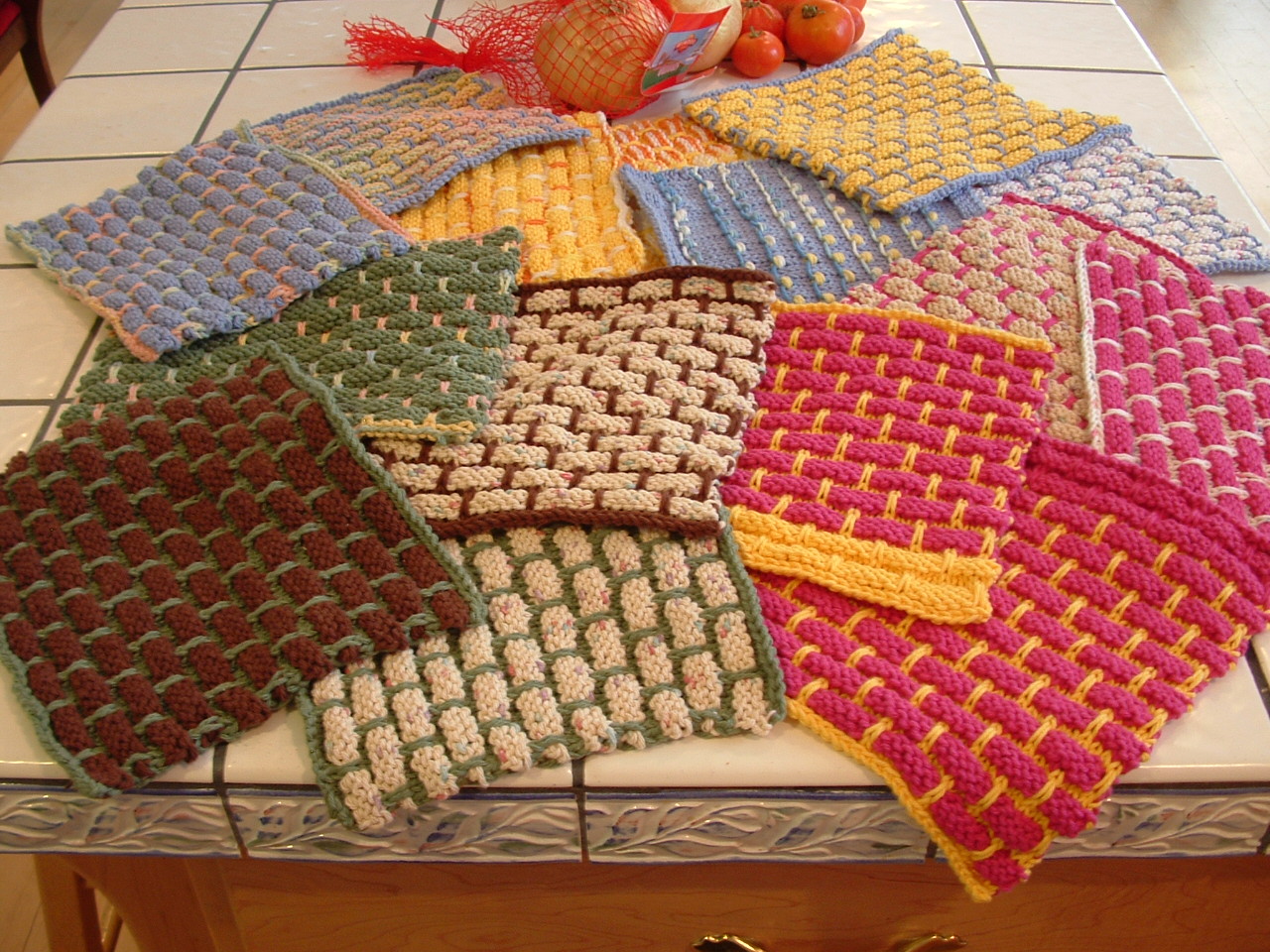The image captures a detailed view of a kitchen island with a ceramic tile countertop. The tiles are off-white with thick grey grout lines, and the edge of the countertop features a raised leaf design that adds a palpable texture. Atop the counter rests a disorderly pile of approximately 12 to 15 knitted placemats, each designed to mimic a brick wall with various colored "bricks" and "mortar." These placemats exhibit a variety of color combinations, including red with yellow accents, brown with green, blue with pink, and raspberry with yellow. Positioned behind the pile of placemats is a red string bag, commonly used for carrying fruit, containing visible small orange fruits that resemble satsumas, as well as a larger item that might be an orange or an onion. Additionally, there are tomatoes and possibly more vegetables scattered further back on the countertop.